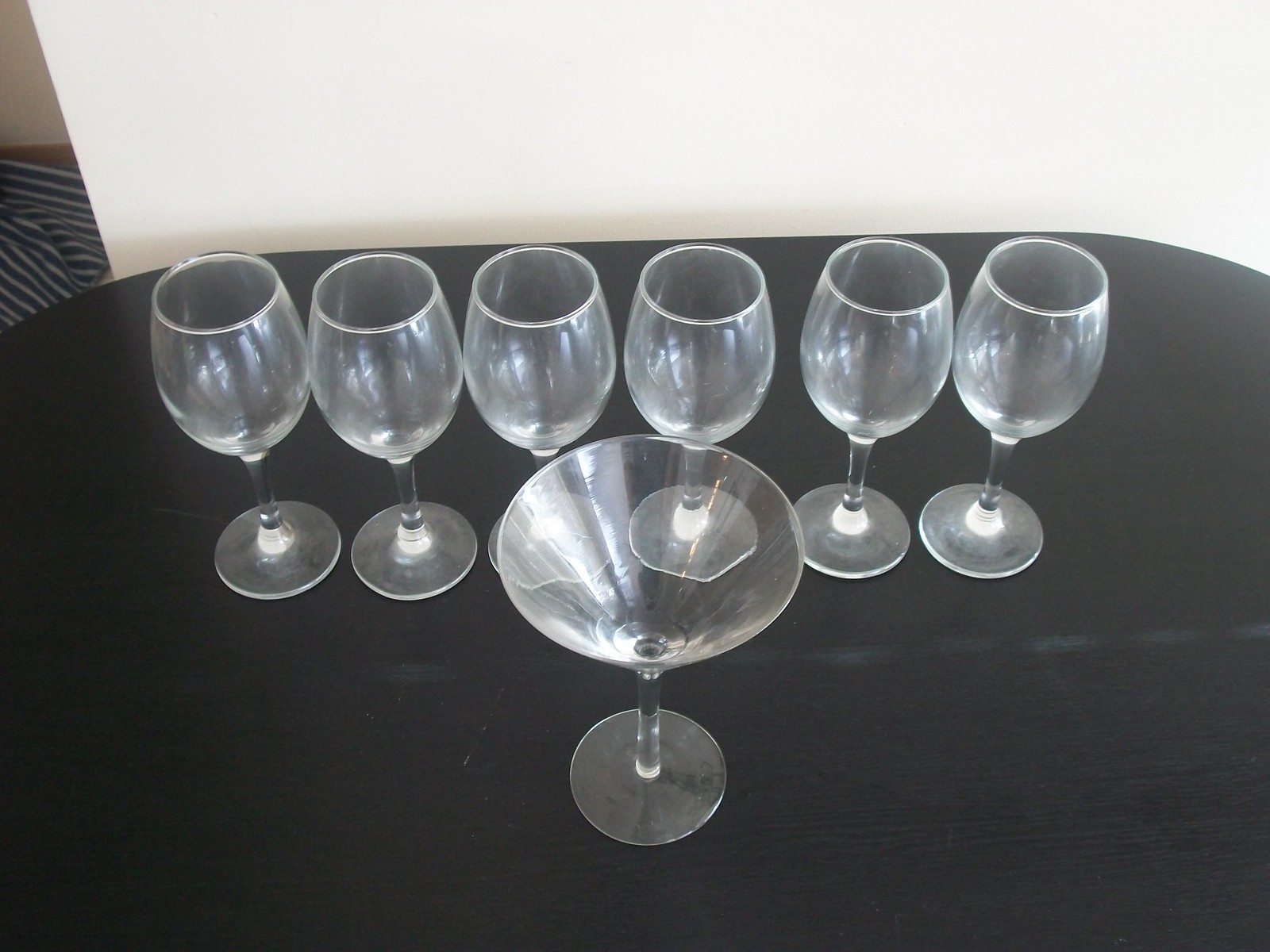In the image, several delicate and elegant glasses are meticulously arranged on a black tabletop. In the foreground, there is a single martini glass with a wide rim that gracefully tapers down to a slender stem and a small round base. Behind it, six tall, tulip-shaped wine glasses are lined up side by side, each with long stems and rounded bases. The glasses are reflective, capturing hints of the surroundings and the light source, which seems to be positioned above or behind the viewer. The background features a white wall and a black and white striped carpet in the top left corner. The scene appears to be a well-prepared setup, possibly getting ready for a party, with all the glasses empty and clean.